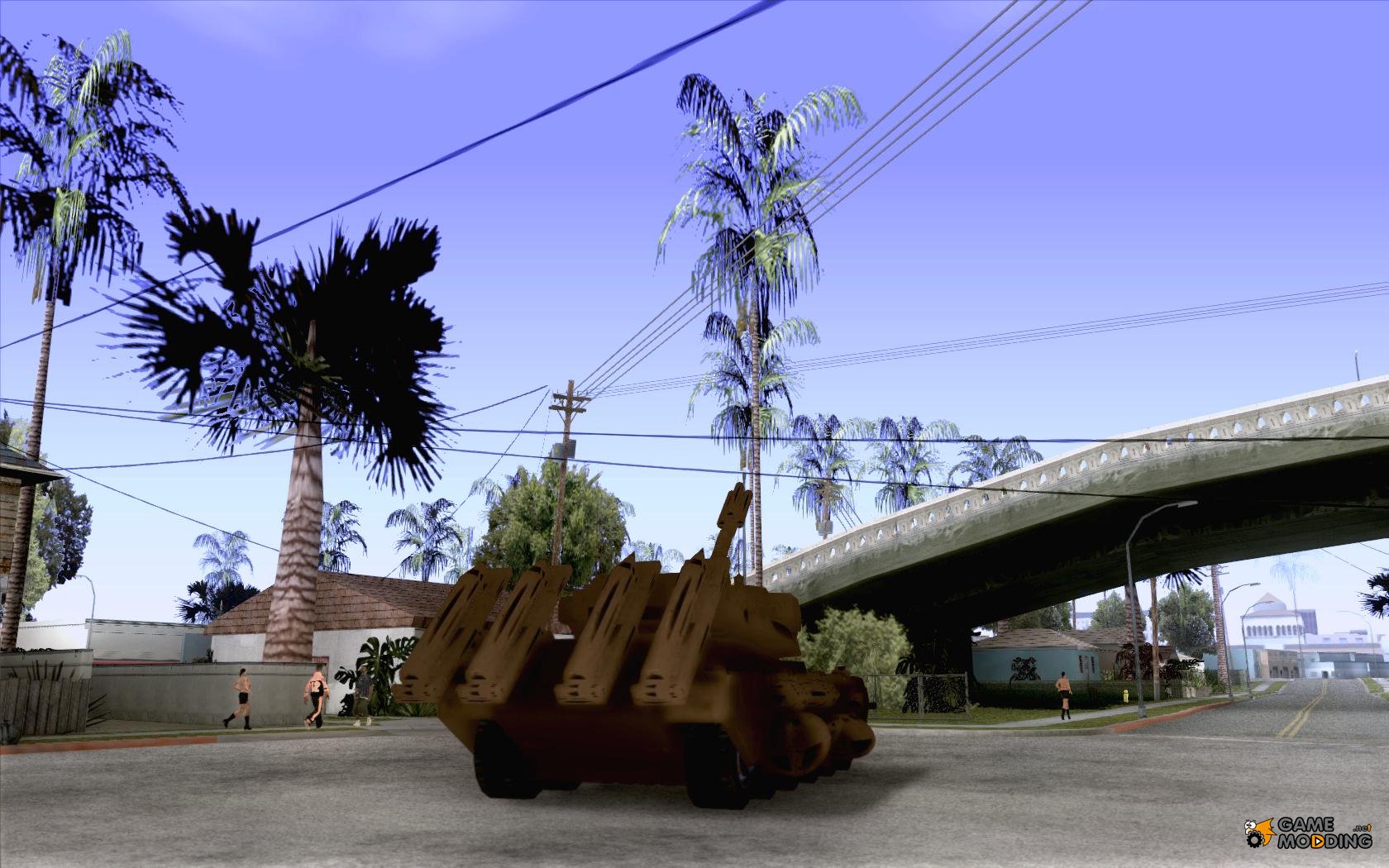This photograph, reminiscent of a scene from the video game Grand Theft Auto, depicts a brightly lit daytime street rendered with pixelated, low-poly geometry. The setting appears to be a cul-de-sac or an intersection, framed by low, single-story homes, including a tan and a blue one, and a scattering of tall palm trees—some with blue fronds, hinting at the computer-generated nature of the image. In the foreground, a dark brown, dirty-colored tank dominates the scene, equipped with four rocket launchers on its back, a tank turret aimed skyward, and tractor treads lining its sides. The overpass bridge above and the numerous power lines crisscrossing the sky contribute to the urban environment. On the sidewalk, three individuals—two walking and one standing—can be seen, dressed in black shorts and socks, with one appearance differing. In the background, large buildings tower over the smaller homes, adding depth to the scene. The bottom right corner of the image features a "Game Modding" logo, confirming its digital origins.